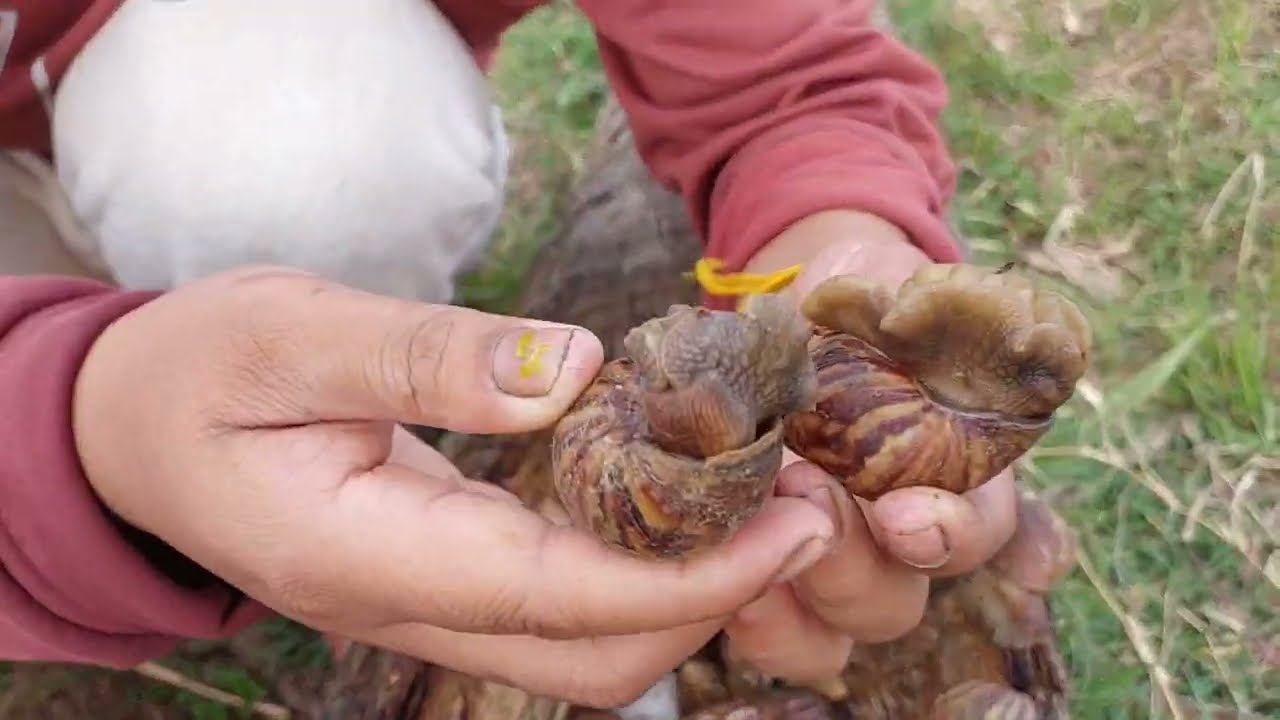The image captures a close-up of a person kneeling outdoors on a grass-covered surface during the daytime. They are dressed in light-colored jeans and a long-sleeved, slightly wrinkled red sweater. Their hands, smudged with gray dirt and showing dirt under the fingernails with a yellow paint stain on the left thumbnail, hold two snails with coiled brown shells. In the background, beneath the person's hands, lies a larger pile of shells on a wooden log. The ground is a mix of green grass blades interspersed with brown, hay-like strands of dead grass and leaves. The scene is devoid of any text and features a vivid palette of colors including white, red, tan, yellow, orange, green, and brown. The image appears to be a personal photograph aimed at capturing an interesting outdoor moment.